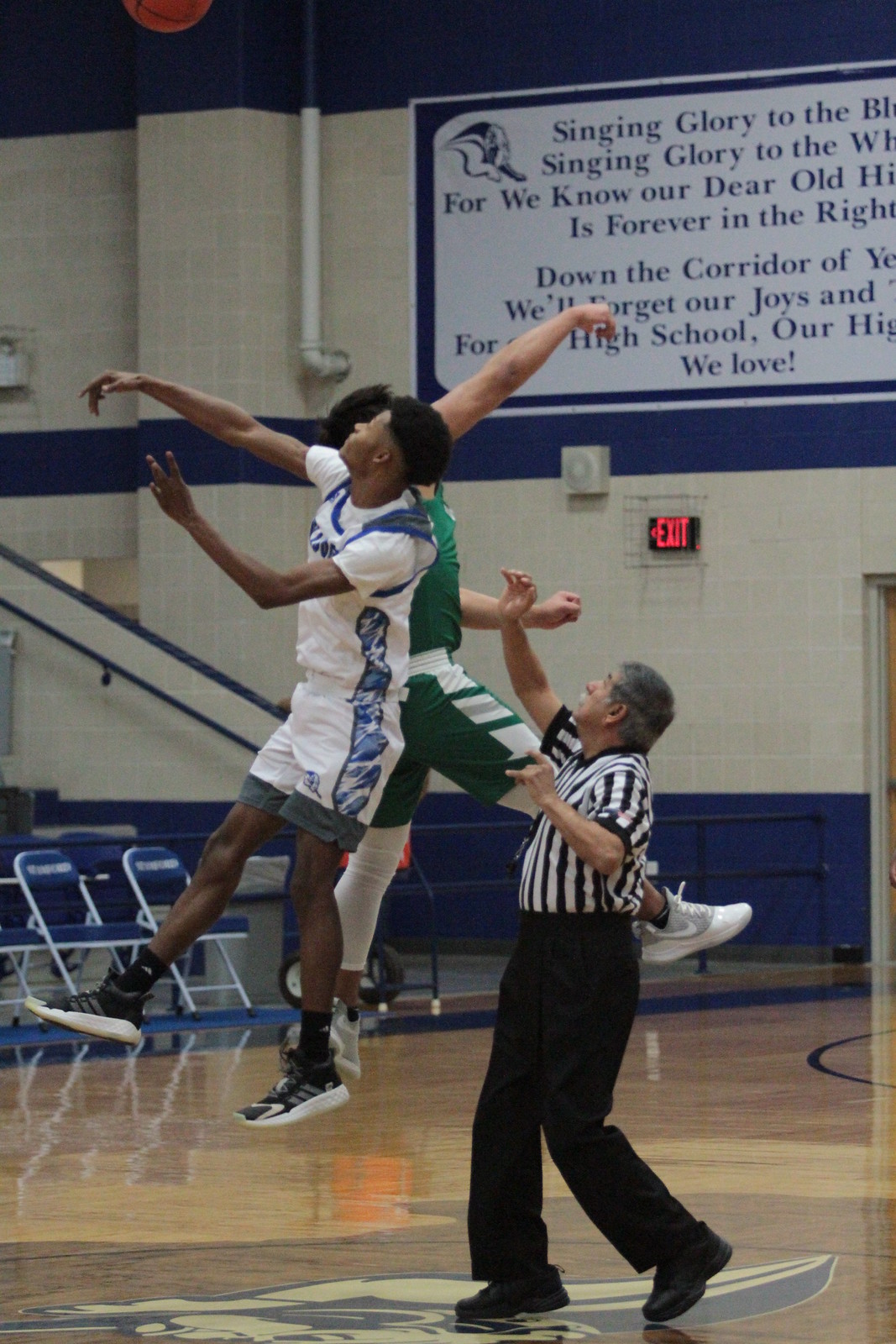In the gymnasium of a high school, an intense moment captures two basketball players and a referee during the tip-off at the start of the game. The hardwood court gleams under the bright lights. To the left, a player donning a white jersey with blue and purple accents leaps high, his black socks and black shoes with white and gray details stark against his crisp white shorts. Opposite him, his rival in midair sports a green and white uniform, with green shorts, white leggings, and white shoes, both of their arms outstretched toward the ball that is just visible at the top edge of the image. Below, the referee, identifiable by his black pants and vertical black-and-white striped shirt, signals the beginning of the match with his right arm extended. His gray hair is a blur as he watches the players ascend. The backdrop features a banner showcasing the school's fight song, hinting at the vibrant school spirit, with the institution's colors, white and blue, reflecting in the gym’s decor and the jerseys of the participants.